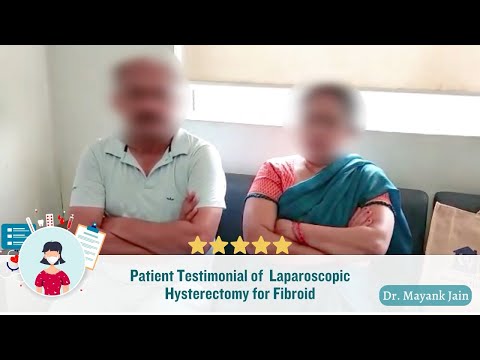The image depicts a man and a woman, both with their faces blurred, seated side by side on a blue bench in an office-like setting. The background is predominantly white, with a window behind them covered by a cream-colored shade pulled nearly to the bottom. They both have their arms crossed, seemingly displaying a non-happy or aggravated demeanor. The woman is dressed in an Indian sari with a blue drape, while the man wears an unbuttoned light green polo shirt. A neighboring blue bench holds a small tote bag. 

At the bottom of the image, a white banner reads "Patient Testimonial of Laparoscopic Hysterectomy for Fibroid," with five yellow stars above indicating a high rating. To the right of the banner, the name "Dr. Mayank Jain" is displayed in white text on a green background. To the left, a circular graphic features a cartoon female figure in a red blouse wearing a face mask, surrounded by illustrations of medical tools like a clipboard, a thermometer, and a heartbeat checker. This visual suggests that the image is part of a testimonial video for Dr. Mayank Jain.